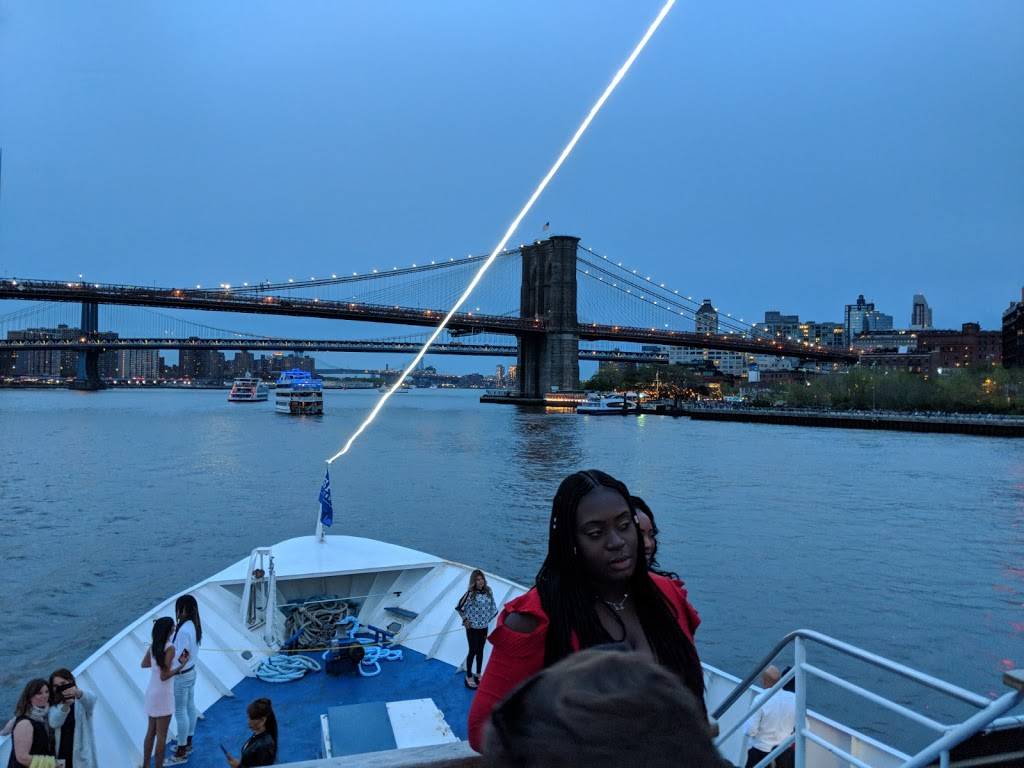In this photograph captured in landscape orientation, the scene is set outdoors during a warm time of the year, likely summer. The primary focus is a boat filled with people, positioned towards the bottom of the image. The passengers, dressed in short sleeves and dresses, suggest a warm evening. The bow of the boat features a blue flag at its tip, with an LED light string extending upward behind the photographer. There are two Black women walking up the stairs, visible on the upper deck, while about six other people are scattered on the lower deck, gazing over the boat's edge.

The river stretches out into the distance under a sky transitioning from daylight to dusk, still holding a twilight blue hue. The middle section of the image is dominated by the water, with several boats dotting the river. A dramatic touch is added by a lightning bolt striking down towards the boat.

In the background, a prominent suspension bridge, adorned with lights, spans the river from left to right. Additional smaller bridges are visible further in the distance. To the right of the bridges, tall city buildings suggest a cityscape reminiscent of New York. The left side of the image also features buildings in the mid-ground. Vegetation, including some small green trees, lines the shoreline off to the right.

The color palette of the photo includes various shades of blue, complemented by whites, yellows, oranges, reds, and pinks, enhancing the overall richness and detail of the scene.